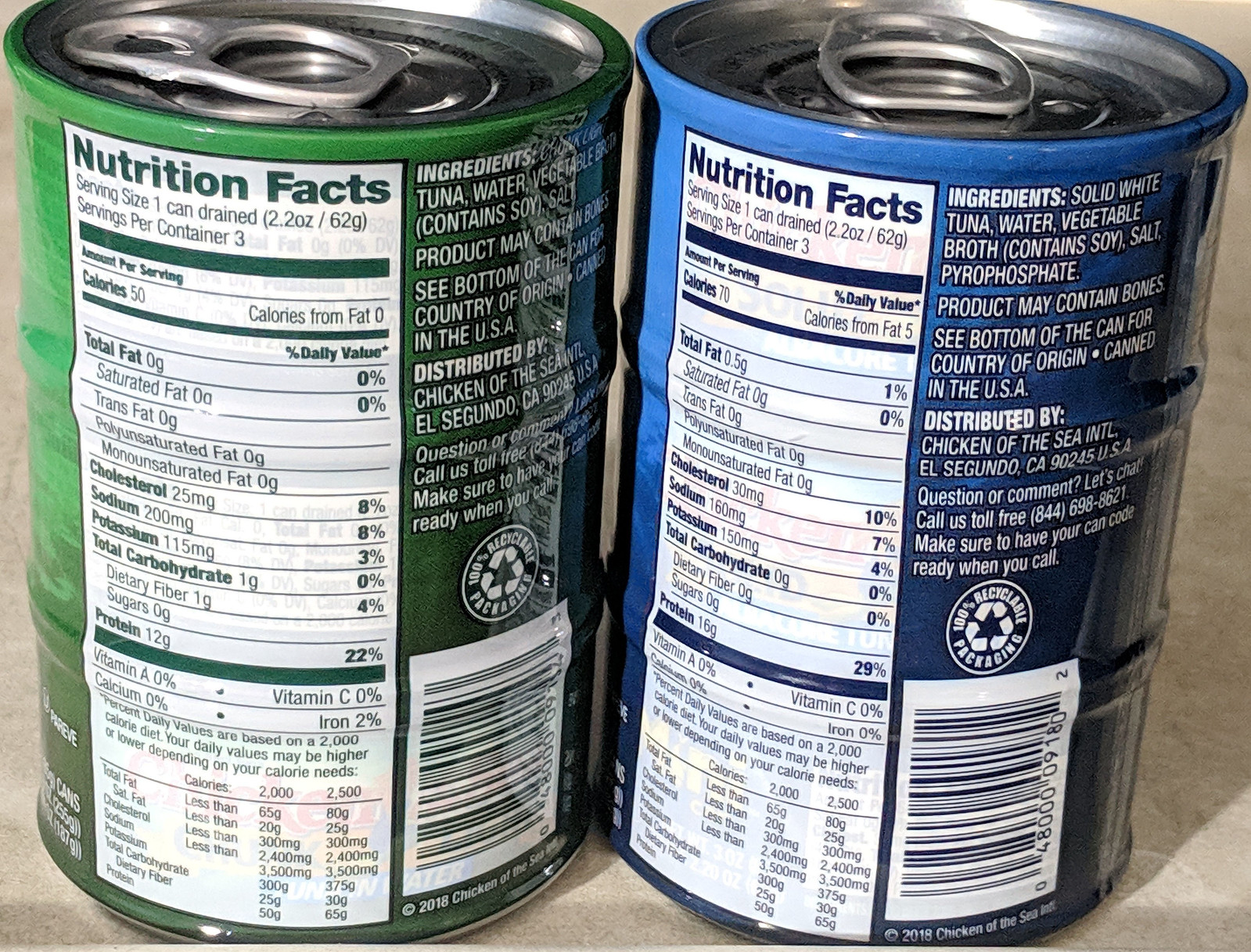The image shows two packs of solid white tuna cans, each pack containing three small cans. One pack features blue labeling, while the other has green. The cans are distributed by Chicken of the Sea and are designed with easy-open pull tabs, eliminating the need for a can opener. The packs are bound together with a plastic wrap. Each can displays nutritional facts, indicating amounts of total fats, saturated fat, trans fat, cholesterol, potassium, total carbohydrates, and protein. The ingredients list reveals that the product may contain bones. Both the blue and green labeled cans include scannable symbols for pricing.